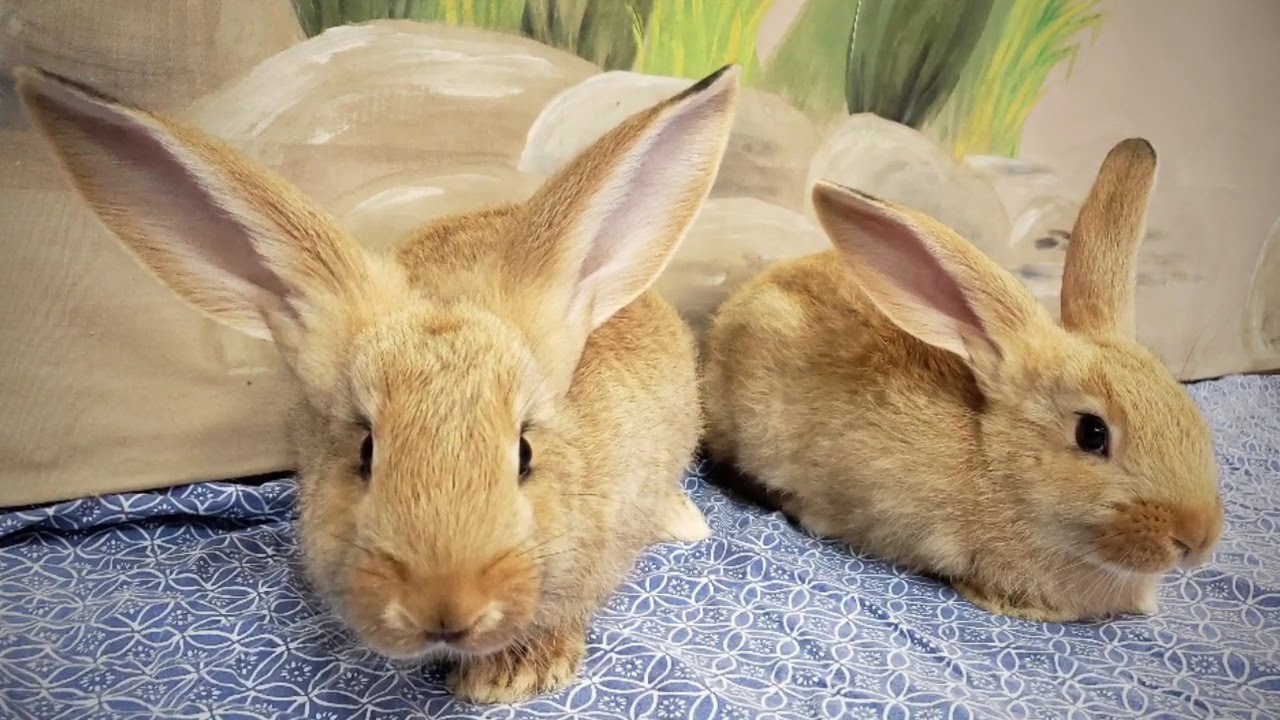In this charming scene, two light tan rabbits with slightly darker noses and eartips are resting close together but not touching, on a blue blanket adorned with white flower-like ovals, creating a peaceful, pastoral setting. The rabbit on the left, with conspicuously large ears, faces directly towards the camera with its front paws visible, showcasing its inquisitive black eyes. The rabbit on the right, with proportionally sized ears, gazes off to the back right, giving a sense of calmness. Behind them is a white wall adorned with a painted backdrop depicting white rocks and an array of greenish plants and grass sprigs, suggesting a whimsical outdoor setting. This intricately painted background enhances the bucolic and serene atmosphere of the image.